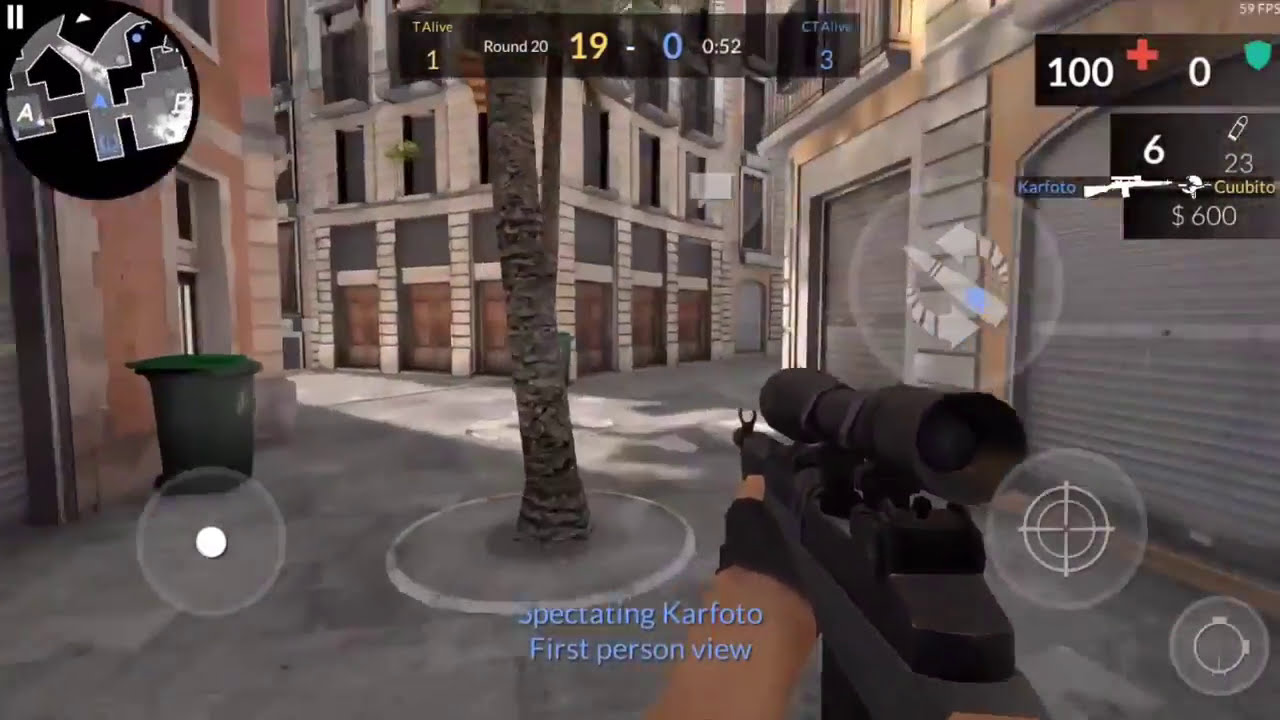The image is a detailed screencap from a first-person shooter video game. The player’s perspective shows them holding a sniper rifle with a large scope, suggesting precision gameplay. The setting is an urban pedestrian street flanked by buildings; prominently, a cream-colored brick building stands center-left, and a red building with a green trash can is to the left. Another structure, also cream-colored, is visible to the right. A tree grows from an asphalt patch with a protective ring at its base, providing a notable central landmark.

An array of HUD (Heads-Up Display) elements overlays the game screen: 
- In the top left, a circular mini-map provides a 2D overview of the player's immediate surroundings.
- Center-top, a scoreboard indicates a score of 19-0 (19 in yellow, 0 in blue), with details including round 20 and status indicating "T alive 1" and "CT alive 3."
- Top right, several stats are displayed: a health meter at 100 with a red cross symbol, armor at 0, 59 FPS (frames per second), ammunition count of 6/23, and total funds of $600 in white font. Beneath, various game status symbols are shown, including a stopwatch icon and crosshairs.
- Bottom center, blue text reads "spectating car photo, first-person view," indicating the player is currently in a spectating mode.

Overall, the combination of vivid scenery details and a rich HUD presents a highly immersive and informative snapshot of a high-stakes in-game moment.